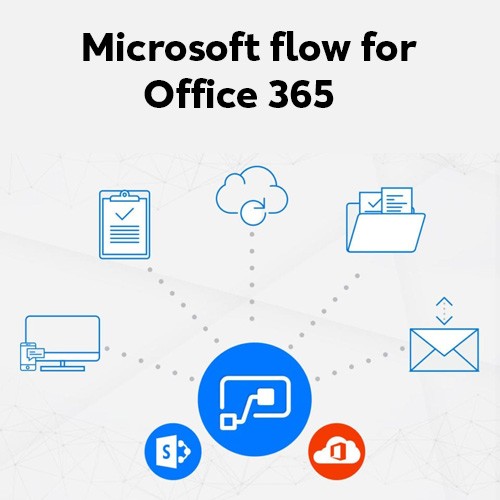The image appears to be an advertisement displayed on a tablet screen, prominently featuring the title "Microsoft Flow for Office 365" in black text at the top center. Below this title are three distinct sections. 

The first section contains a blue circle with a white background and blue writing, though the specific text is unreadable. The second section, also unreadable, is adjacent to the first.

In the middle of the page, there's a larger blue button with white text, symbolizing an interaction of devices, possibly a connection or synchronization, illustrated by icons resembling plugs or connectors.

The bottom right section features a red background with a white cloud, likely associated with the Opera browser logo, indicating integration with cloud services. 

Extending from the large blue button are dotted lines leading to various icons, each signifying different Office 365 functionalities: a computer and cell phone representing device compatibility, a clipboard for task management, a cloud for storage, a folder with documents for file organization, and an envelope symbol for email.

This comprehensive layout effectively highlights the interconnected features of Microsoft Flow within Office 365's ecosystem.